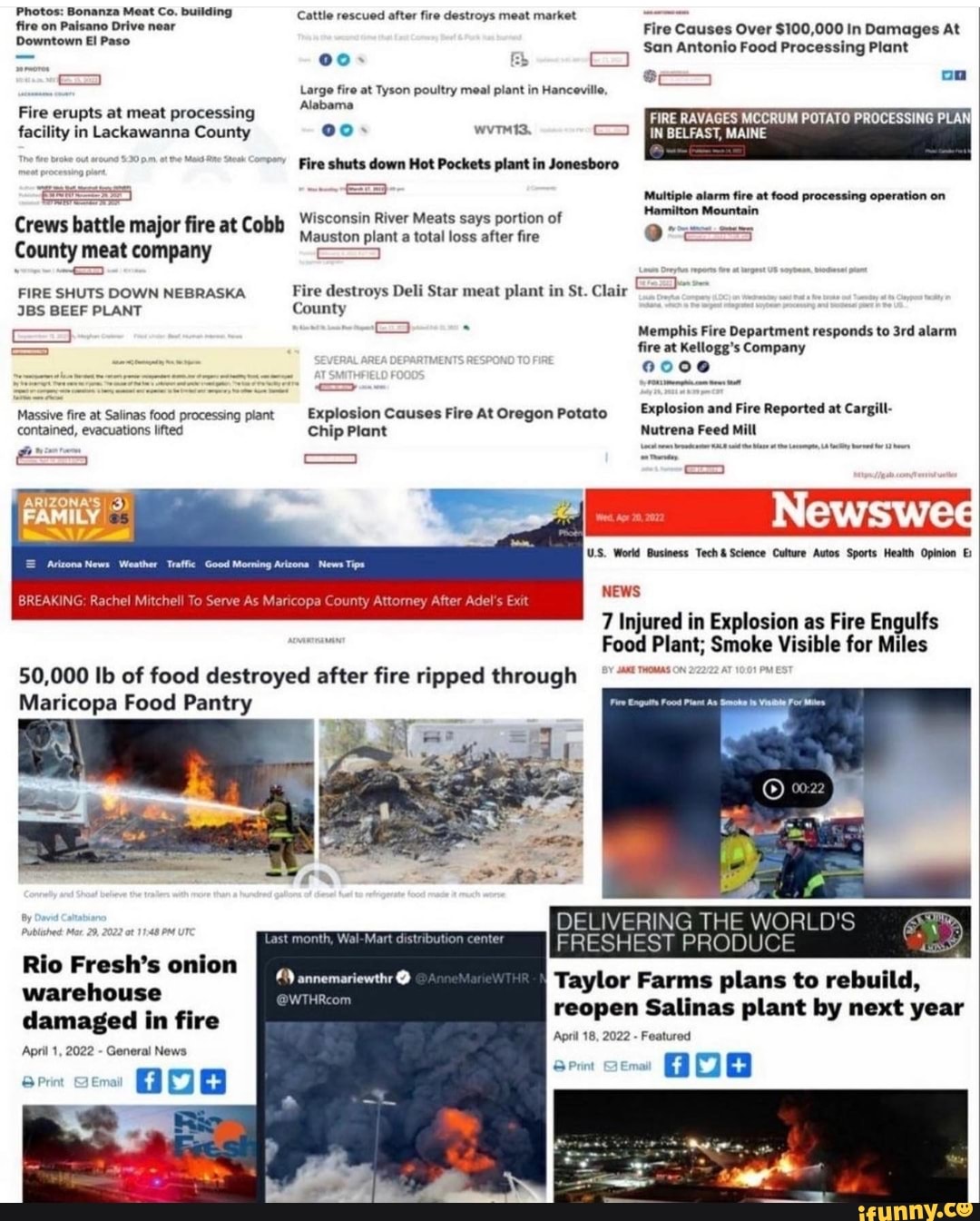The image showcases a collage of news articles and website snippets, meticulously pieced together to form a comprehensive visual. Each piece of the collage contains headlines and excerpts from various news sources such as Newsweek, detailing multiple incidents of fires at food processing facilities. Highlighting the severity of these events, red rectangles encircle specific areas within the image to draw attention to key incidents.

At the top, one headline reads, "Fire erupts at meat processing facility in Lackawanna County," while adjacent snippets report, "Crews battle major fire at Cobb County Meat Company," and "Fire shuts down Hot Pockets plant in Jonesboro." Additional headlines reveal more distressing news: "Fire destroys Deli Star meat plant in St. Clair County," and "Explosion causes fire at Oregon potato chip plant."

Other notable incidents include a headline stating, "Fire causes over $100,000 in damages at San Antonio food processing plant." The image further details a fire that led to the destruction of 50,000 pounds of food at Maricopa Food Pantry, and another severe fire that injured seven individuals and generated smoke visible for miles.

Structured in a descending order, the collage methodically lists numerous fire incidents across various food processing plants, forming a troubling narrative of frequent and costly occurrences in the industry.